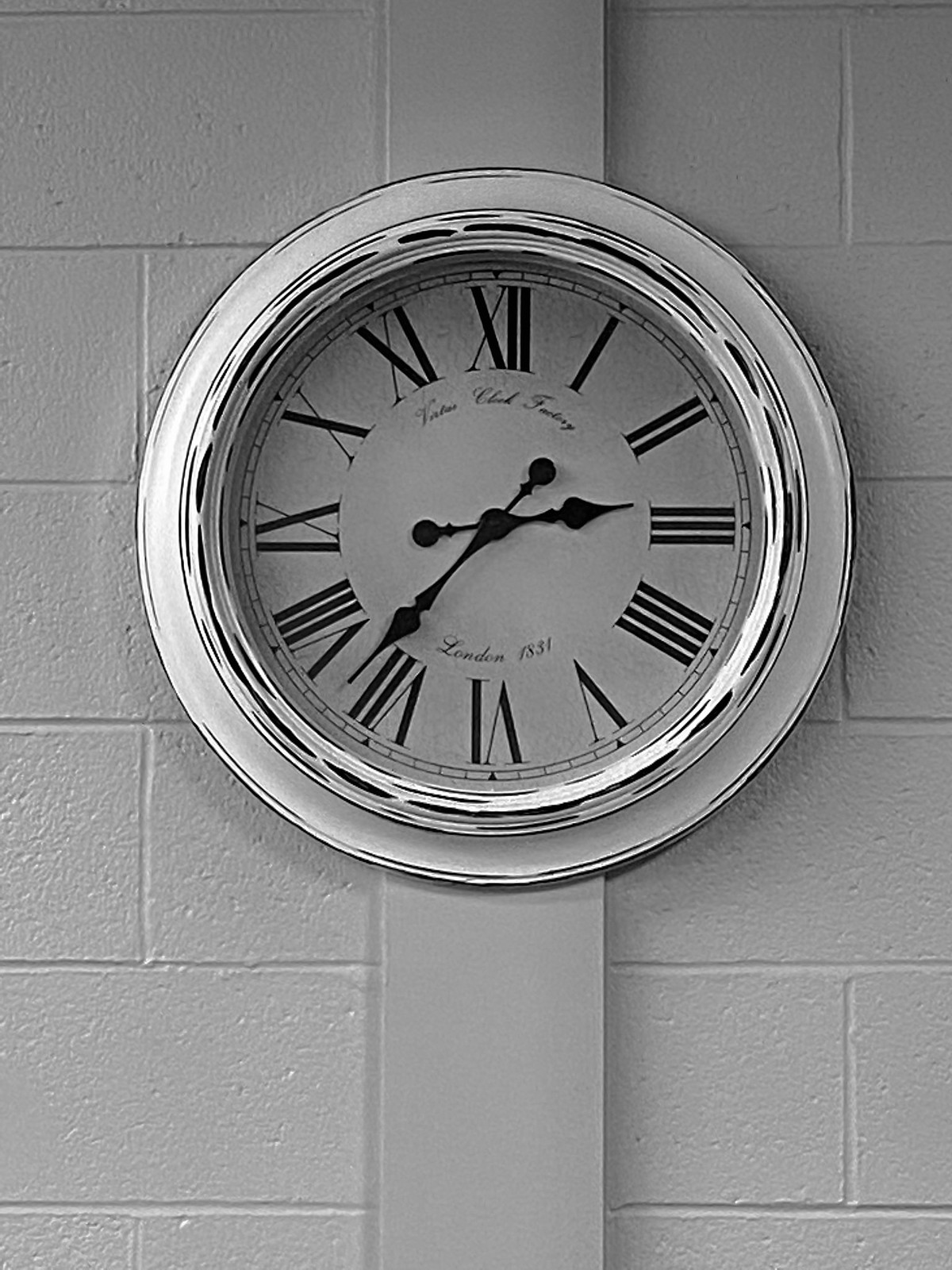In this detailed black-and-white photograph, a beautifully crafted clock hangs prominently on what appears to be an off-white concrete block wall, shaped to resemble bricks. The clock has a round, silver-colored frame that is beveled inward towards the center, causing the Roman numeral markers to look slightly recessed. The clock face itself is a light, off-white color, contrasting elegantly with the bold black Roman numerals that encircle it. The time display reads almost 2:40, indicated by black metal hands with tiny balls at the base and arrow-shaped tips. In the center, cursive writing reads "Veritas Clock Factory," and near the bottom, the text "London 1831" is inscribed. The entire piece exudes a timeless, classic charm, accentuated by the reflective gleam of its silver elements and the meticulous design of its black hands and Roman numerals. The wall behind the clock has a neat, rectangular etching that mimics the appearance of bricks, enhancing the vintage aesthetic of the setting.